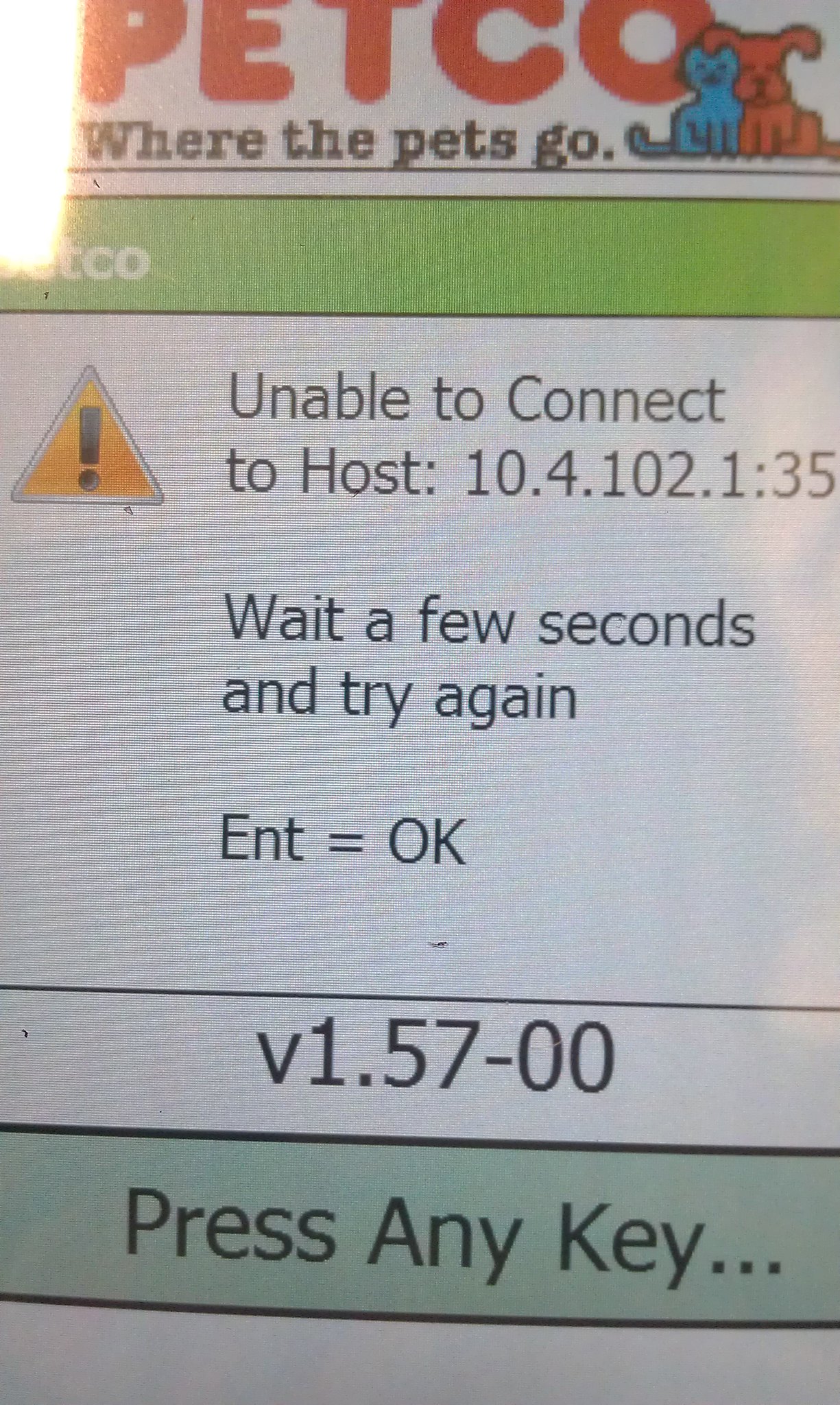The image depicts a digital screen with various prominent details. At the top center, there is the Petco logo, featuring "Petco" in big red letters against a white background, partially obscured by a glare. Below the logo, the slogan "where the pets go." is displayed in black font. To the right of the slogan, the Petco symbol is visible, featuring a blue kitten and a red dog nestled together. Underneath this, a green rectangular area contains the faded white letters "Petco" on the left side.

Below this section, a white background displays two separate parts of text. The first part states, in black letters, "unable to connect to host 10.4.102.1:35." To the left of this text, there is a large yellow triangle with a black exclamation point. Underneath this message, it says "wait a few seconds and try again. ENT equals okay." Further down, within another white section, "V1.57-00" is printed in black letters. Towards the bottom of the image, another green area displays the text "press any key..." in black font. Finally, the lower part of the image is a plain white section.